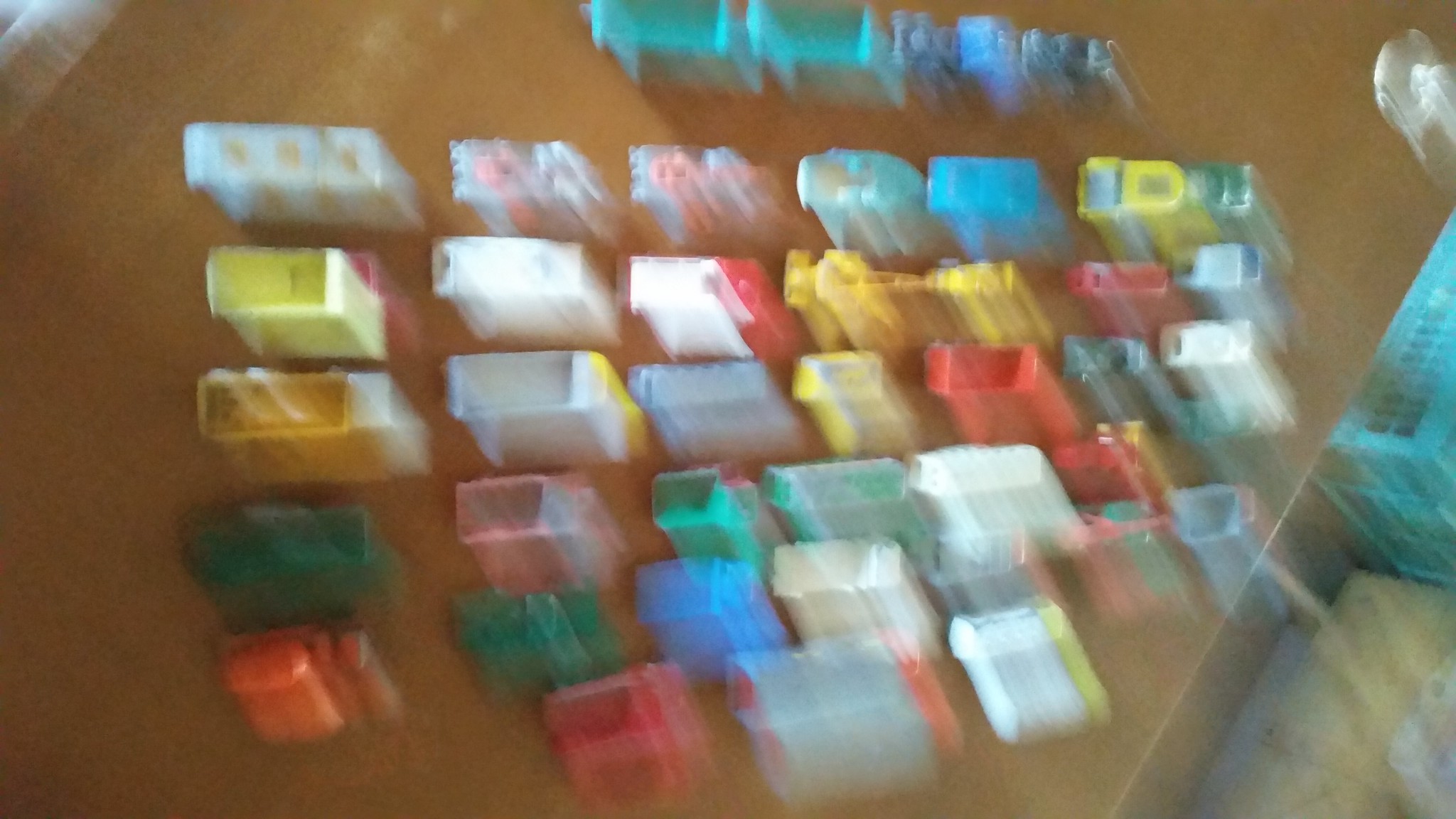On a wooden table, an array of small rectangular containers, reminiscent of Tic-Tac boxes but clearly not, are meticulously arranged. Each container, potentially housing components for a technological device, varies in orientation with some aligned horizontally and others vertically. There are approximately 15 to 20 of these containers, organized neatly in rows. To the right of this orderly display, a green basket can be seen, adding a touch of color to the otherwise neutral-toned setup. The scene suggests a workspace dedicated to sorting or assembling technology parts.